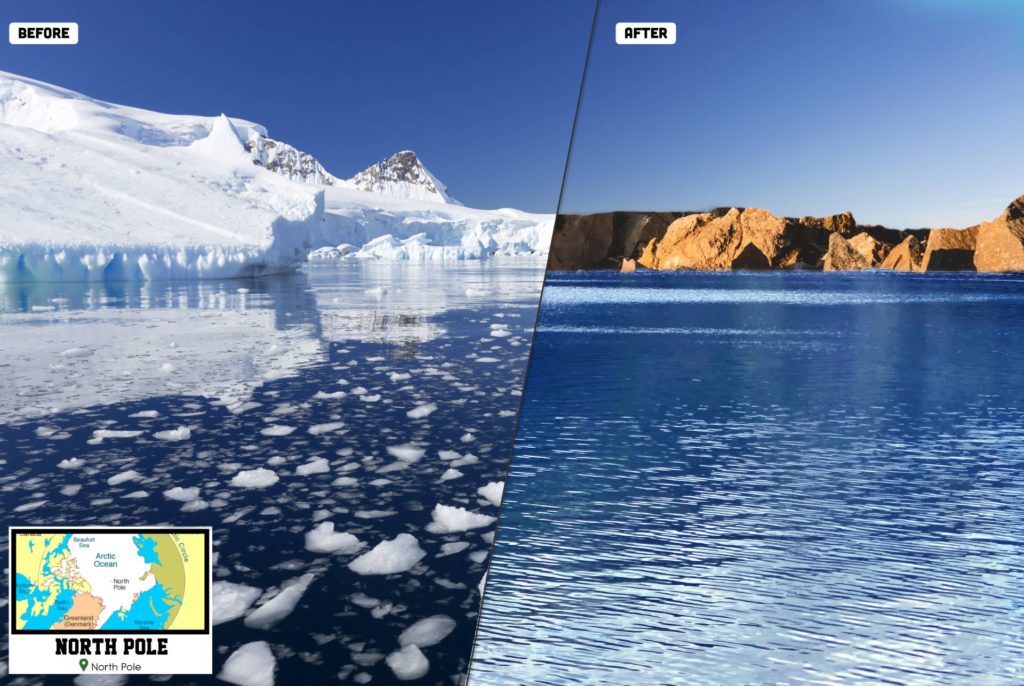This outdoor, photographic image is a powerful before-and-after depiction of glacial retreat, highlighting the impact of climate change. The photo is split into two vertical halves. The left side titled "BEFORE" in bold black letters on a white background shows a majestic scene of massive ice glaciers and chunks of floating ice under a bright blue sky. The water int he "before" is a deep, darker blue. The right side labeled "AFTER" starkly contrasts with an absence of glaciers and floating ice, replaced by barren, brown rock cliffs and a lighter blue expanse of water, still under a bright blue sky. In the bottom left corner, a map of the Arctic region includes labels like "North Pole," "Arctic Ocean," "Greenland," and "Arctic Circle," although some parts are blurred and hard to read. The visual transformation from a frozen, ice-covered landscape to a desolate, ice-free environment underscores the severe effects of climate change.